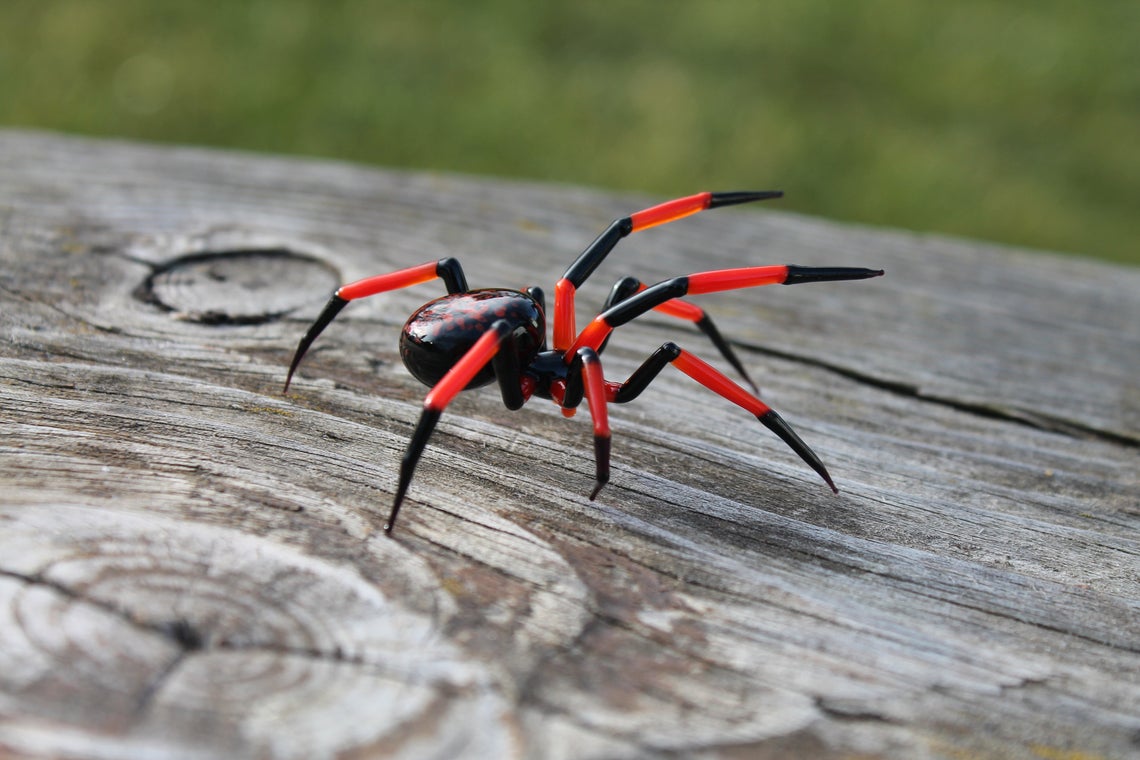This is a close-up, highly detailed image of a large, intimidating spider crawling across a weathered wooden picnic table, likely situated in a park. The spider's legs exhibit an alternating pattern of black and bright red segments, while its glossy black body is adorned with various red to orange markings, making it visually striking. Captured from the side, the spider's bulbous, round body stands out prominently, and its size suggests that it is several inches across. Its front two legs are raised in the air, as if sensing the environment ahead. The background of the image is blurred, displaying a green hue indicative of grass, emphasizing the hyper-focused nature of the spider. Despite a slight ambiguity about its true nature—whether a dangerous, potentially poisonous creature or an eerily lifelike plastic model—the spider's menacing appearance makes it something one would instinctively avoid.